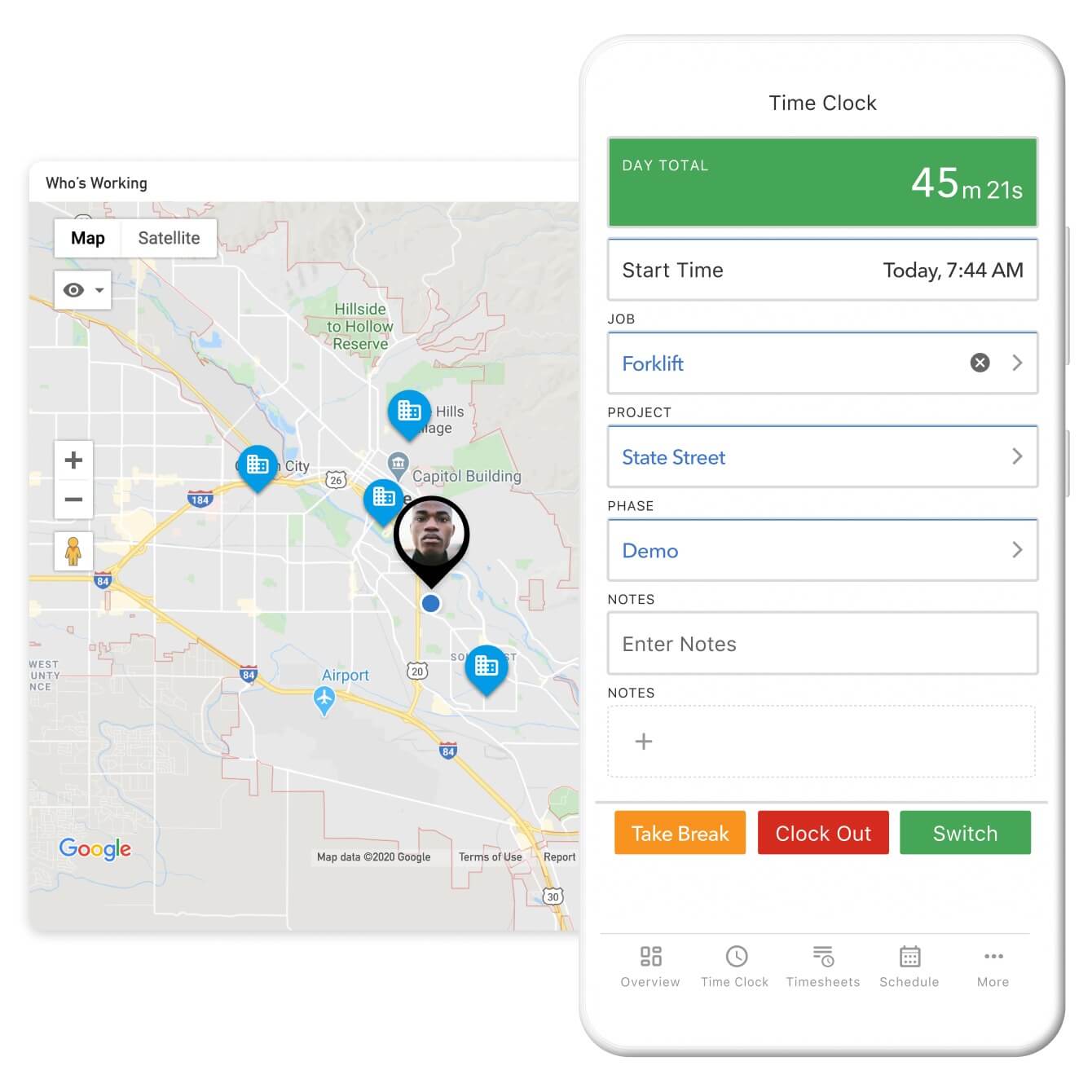The screenshot features a simulated display of a webpage or application interface, likely intended as a demonstration or advertisement. The image appears to be a composite shot, combining various elements to provide an overview of the app's functionality.

In the background, there is a map with a search box labeled "Who's working." The map includes several interactive icons and features. On one side, a text box offers the option to switch between "Map" and "Satellite" views. There is also an information icon, a drop-down menu, and zoom controls represented by plus and minus signs. The map displays multiple blue location markers, one of which features the image of a male individual. Notable landmarks on the map mentioned include "Hillside to Hollow Reserve" and an airport, although the specific city is not identified.

In the foreground, a digital image of a white smartphone is superimposed on top of the map. The phone screen shows a detailed interface with various data points:
- A heading that displays "Time Clock" and the total time recorded as "45m 21s."
- The start time for the current day, noted as "7:44 AM."
- Job details such as "Forklift Project" and "State Street Phase Demo."
- An area for entering notes and several function buttons at the bottom of the screen.

Overall, the image appears to serve as a promotional demonstration of an app designed to track work time and project details, utilizing both map-based and phone interface elements.